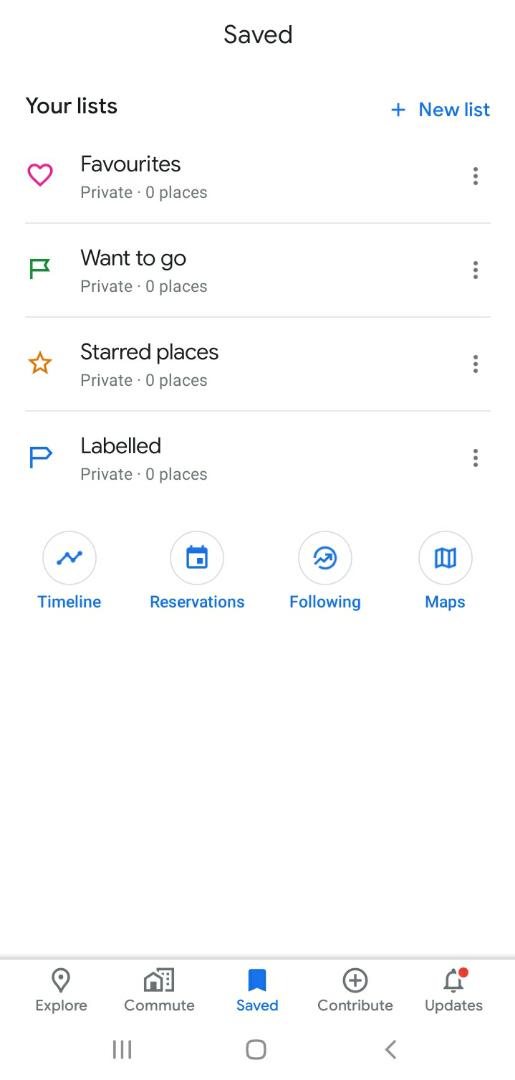The image is a vertically rectangular screenshot taken from a cell phone, displayed against a white background. At the very top-center, the text "Saved" is prominently visible. Moving downward, on the left side, the heading "Your lists" is displayed, while on the right, in blue text, the option "＋ New list" is visible. Below the heading "Your lists," and slightly indented to the right, there are several icons and their corresponding categories:

1. A pink heart icon with the label "Favorites," marked as private, and indicating "0 places."
2. A green flag icon with the label "Want to go," also marked private, with "0 places."
3. A gold star icon labeled "Starred places," private, with "0 places."
4. A blue 'P' icon labeled "Labeled," private, and "0 places."

Beneath these categories, there are four circular buttons horizontally aligned, each featuring an icon in the center and a label below:
- "Timeline"
- "Reservations"
- "Following"
- "Maps"

Following this section, there is an area comprising a plain white background. At the very bottom of the image, a horizontal row of icons with their descriptions is shown. These icons and labels include:
- "Explore"
- "Commute"
- "Saved"
- "Contribute"
- "Updates"

Overall, the screenshot details various list categories and navigation options available within a specific app interface.